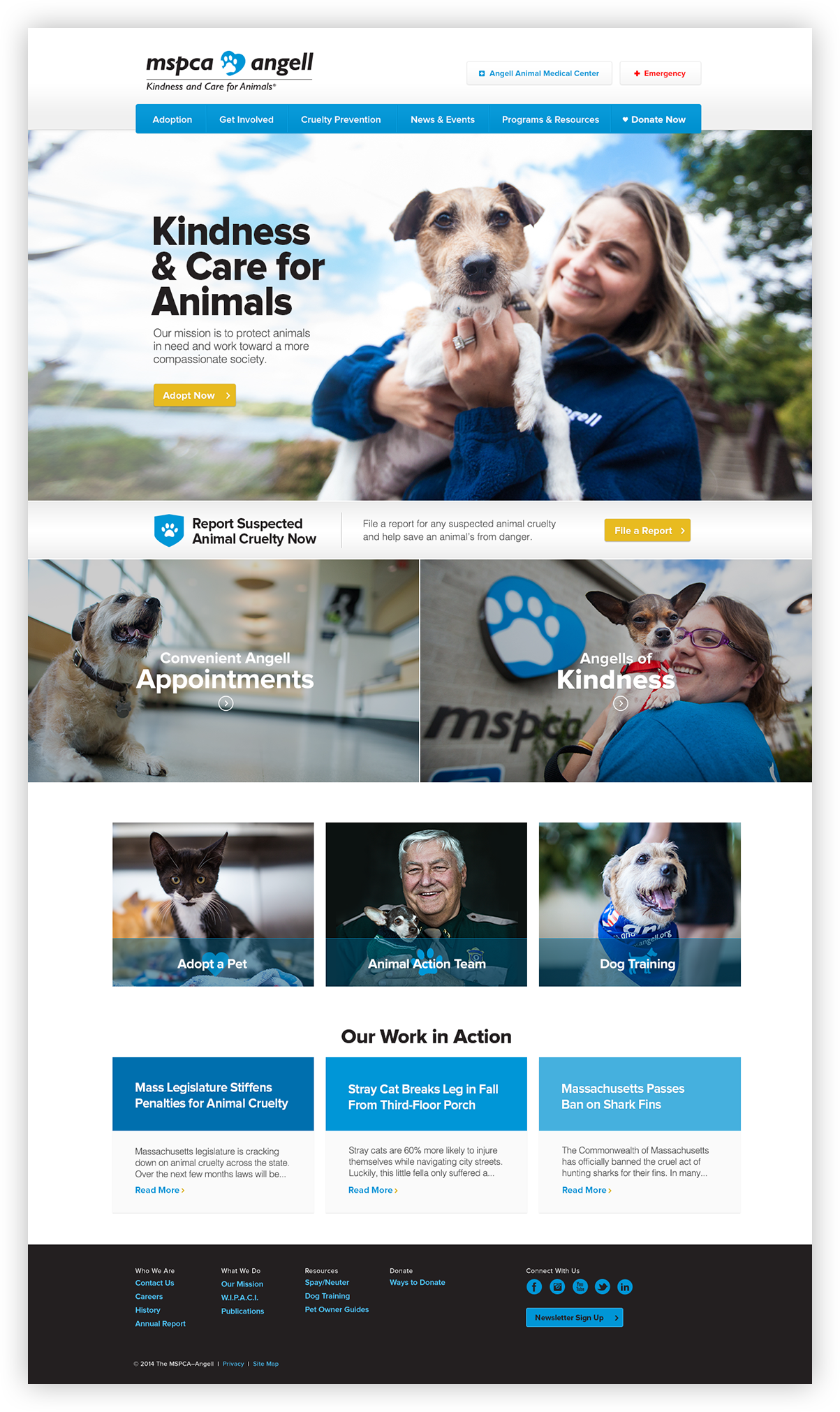The webpage is a detailed overview of the MSPCA (Massachusetts Society for the Prevention of Cruelty to Animals) ANGEL, highlighting their commitment to kindness and care for animals. 

At the top, there are prominent buttons labeled "ANGELI," "Animals and Kinder," and "Emergency," designed for quick and easy access. Below this header, a blue bar showcases multiple navigational options, including "Adoption," "Get Involved," "Cruelty Prevention," "News and Events," "Programs and Resources," and "Donate Now," offering a comprehensive guide for those interested in various forms of support and involvement.

The main section features a heartwarming image of a woman holding a carrier with a brown and white dog, characterized by its dark brown ears and a light brown patch on its head. The woman has dirty blonde hair. 

Key banners beneath this snapshot include:
- "Kindness and Care for Animals": A mission statement aligning with their goal of fostering a compassionate society and protecting animals in need.
- "Adopt Now": Highlighted in a yellow bar to encourage immediate action.
- "Report Suspected Animal Cruelty Now": A call to action for viewers to file reports about suspected cruelty, emphasizing the role of the public in safeguarding animals.
- "Convenient ANGEL Appointments": Featuring an image of a shaggy dog looking up expectantly, likely indicating the ease of setting appointments.
- "ANGELs of Kindness": Depicting a woman holding a small, tired-looking chihuahua, this banner underscores their compassionate care services.
- "Adopt a Pet": Showcasing a black and white tuxedo-haired kitten, encouraging pet adoptions.
- "Animal Action Team": Illustrated by an older man holding a chihuahua, indicating a proactive team involvement.
- "Dog Training": Displaying a well-trained dog in uniform, this section promotes their training programs.

At the bottom, there are sections titled "Artwork in Action" and news highlights such as "Mass Legislation Stiffens Penalties for Animal Cruelty," "Stray Cat Breaks Leg in Fall from a Third Floor Porch," and "Massachusetts Press Banned on Shark Fins," providing updates on advocacy and legislative efforts. 

The footer provides additional resources and information about the organization's mission, history, career opportunities, contact details, and ways to donate. Overall, the webpage serves as a comprehensive guide to the MSPCA ANGEL's offerings, initiatives, and opportunities for community engagement in animal welfare.